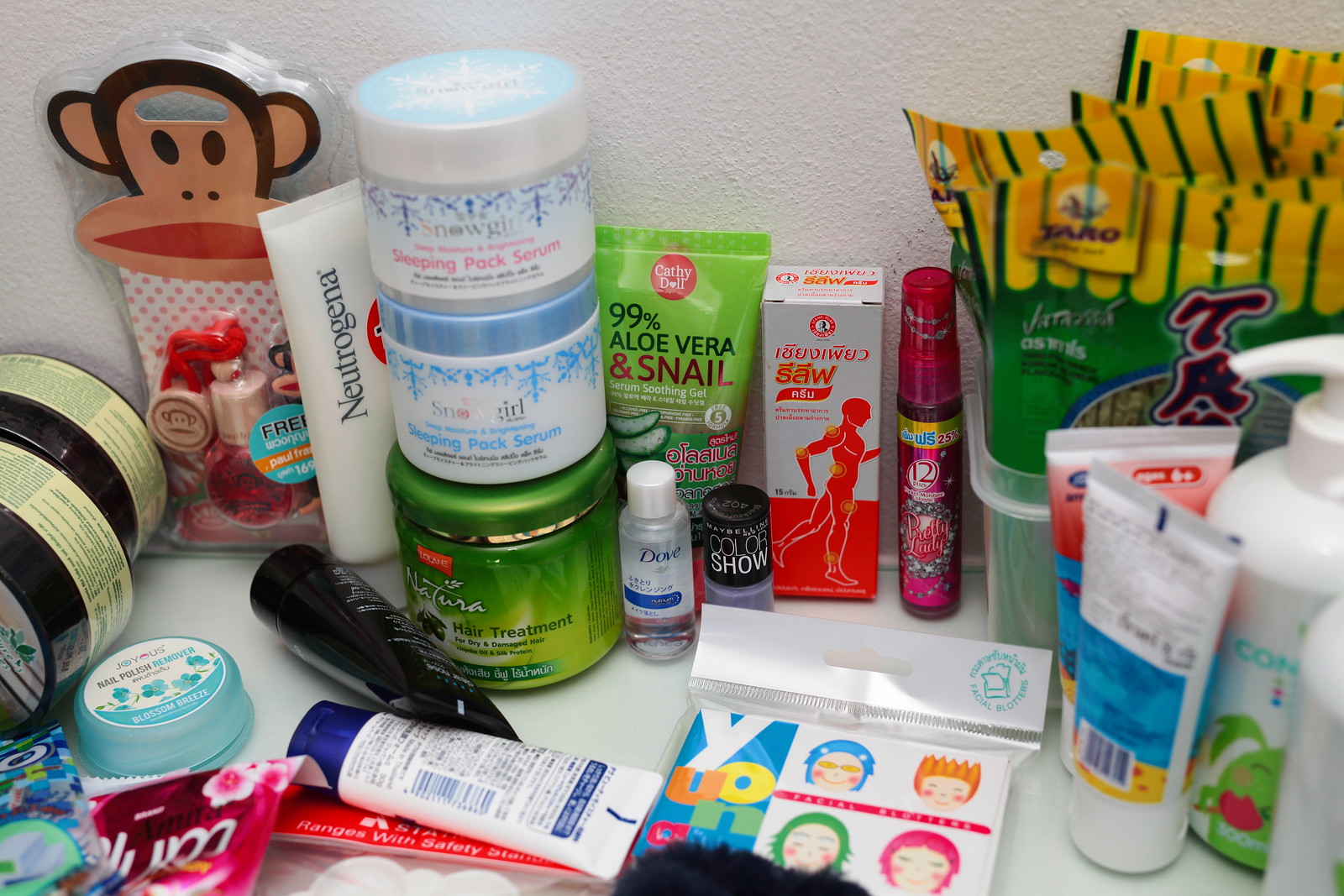This is a vibrant color photograph showcasing an assortment of beauty products meticulously arranged on a pristine white surface with a white wall as the background. At the forefront, there is a Paul Frank themed beauty kit featuring the iconic monkey logo prominently displayed at the top of the packet. The contents of this packet remain obscured. Surrounding it are various containers including green jars with black lids, and a small blue bottle labeled "Joyous Nail Polish Remover Blossom Breeze." Adjacent to these is a white tube capped with blue, its label concealed from view, and a black tube lying on its side.

Prominently displayed is a white tube with "Neutrogena" printed along its side. There is also an intriguing stack of three jars: the topmost one is white adorned with a blue lid bearing the inscription "Snow Girl Sleeping Pack Serum," the jar beneath shares a similar inscription but with a darker blue lid, and the largest jar at the bottom is green, emblazoned with "Natura Hair Treatment for Dry and Damaged Hair."

Further to the display is a green tube labeled "Cathy Doll 99% Aloe Vera and Snail Serum Soothing Gel," and a small clear bottle branded Dove with Japanese writing. A lavender-hued nail polish bottle marked "Maybelline Color Show" stands out adjacent to a white box illustrating a profile of a man walking towards the right, with various parts of his body circled; the label is in a foreign language. Nearby is a pink spray bottle labeled "Pretty Lady" and a plastic bin filled with green and yellow packages of indeterminate contents.

To the far right, the image features more unidentified tubes, culminating with an intriguing item in a plastic bag decorated with four cartoon faces. This detailed arrangement of beauty paraphernalia is diverse and visually engaging, depicting a broad spectrum of personal care products.